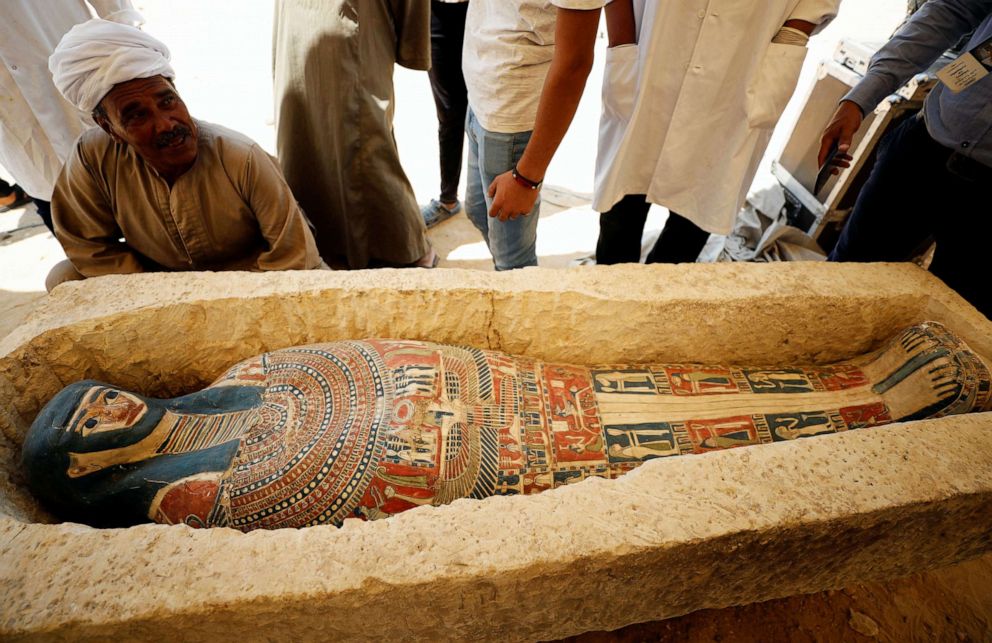The image depicts an ancient Egyptian sarcophagus on display, most likely associated with a pharaoh. The outer sarcophagus is made of a light yellow or beige-brown stone with a rectangular carved-out center. Inside, a highly detailed, human-shaped casket is visible. The casket is adorned with various Egyptian hieroglyphics and imagery, featuring a painted face with black hair cascading down the shoulders, black eyes, red lips, and painted feet with blue sandals. The sarcophagus cover is rich in colors such as gold, blue, red, green, and white, showcasing elaborate patterns and hieroglyphics.

Surrounding the sarcophagus are several people who appear to be archaeologists or visitors, although their heads are mostly cropped out of the photograph. One prominent figure, bending down in front of the sarcophagus, is a man with a dark complexion wearing a white turban, a brown button-down long-sleeved shirt, and sporting a mustache. He seems to be engaged in conversation with another individual. Additional observers can be seen, including a person in a blue shirt and jeans with a name tag and a black cell phone, and others in lab coats and varied attire. The scene is brightly lit, suggesting they might be under a tent, and there's visible brown sandy dirt in one corner, indicating a potential excavation site.